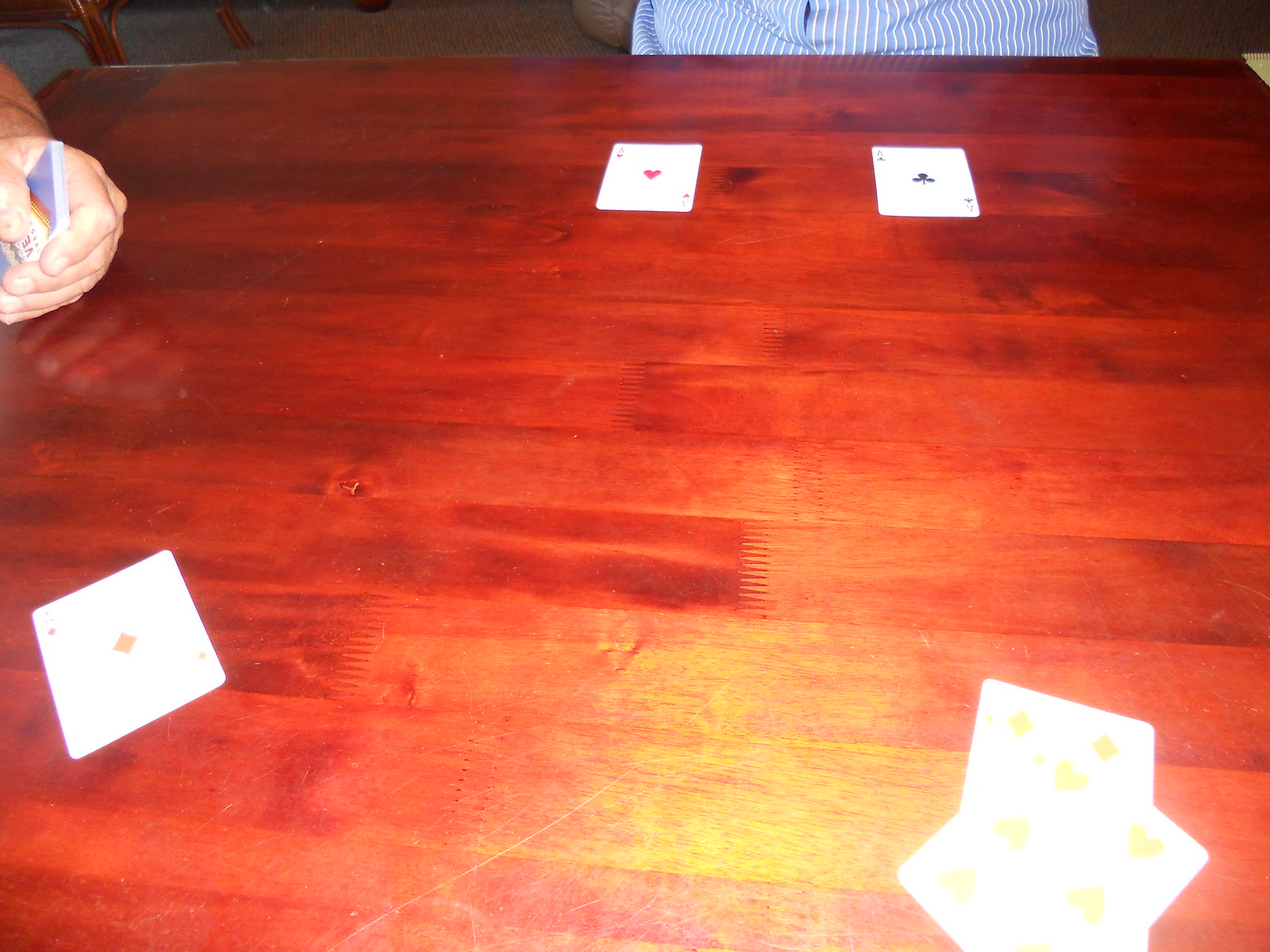This photo, seemingly taken with a cell phone and a flash, captures a moment in a card game among three players. The player directly opposing the photographer's point of view is wearing a blue shirt with vertical white stripes, barely visible at the bottom edge of the frame. On the table in front of this player are the Ace of Clubs and the Ace of Hearts, both positioned with their faces directed toward the camera. To the left, another participant shows only their left hand, holding a bunch of face-down cards, while an Ace of Diamonds lies directly in front of them. On the right side, a player has two cards, one distinctly the Six of Hearts and the other appears to be the Six of Diamonds, though it's partially obscured, making it difficult to be certain. The game is being played on a table made of polished reddish wood, possibly cherry, standing on carpet, as indicated by a small visible section at the back of the photo. An additional wooden leg is faintly visible to the side. The camera angle and the card orientations suggest that all the cards are positioned facing the person taking the picture.